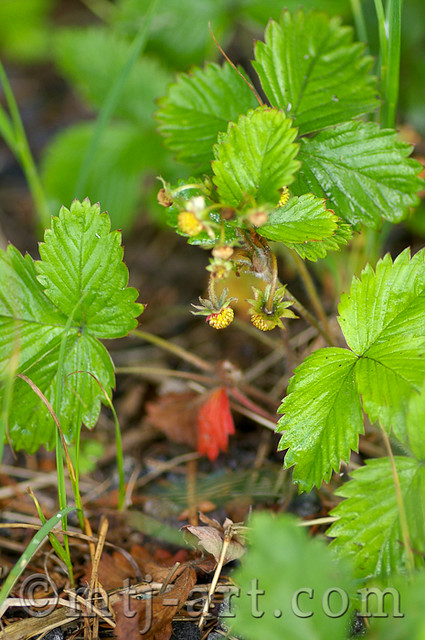A close-up photograph, likely magnified, captures a vibrant strawberry plant bathed in natural moisture, suggesting recent rain or a damp atmosphere. The main focal point of the image is a cluster of green leaves, arranged in groups of three, each glistening with droplets of water. Nestled within this foliage are five to seven budding strawberries, hinting at the promise of future fruit. Scattered among the plant are interspersed twigs of grass and a dead leaf tinged with brown and red, enhancing the natural setting. The background, slightly blurred, reveals a mix of decaying leaves and debris, illustrating a typical outdoor environment. The image is marked with a discreet watermark reading "copyright mtj-art.com" at the bottom.